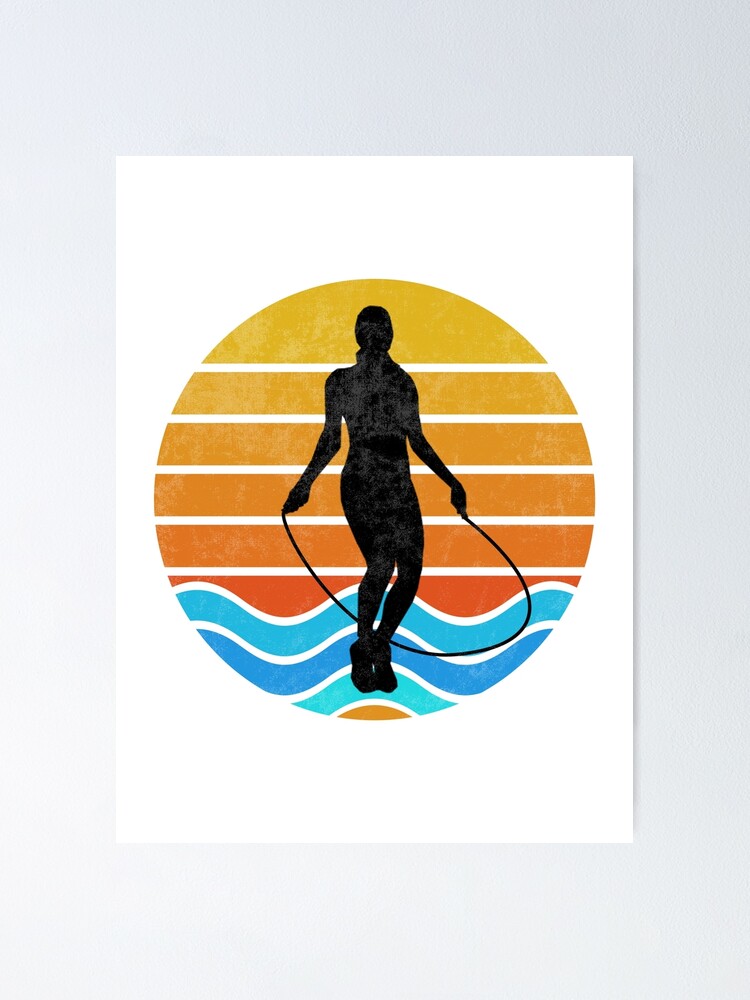The image depicts a modernistic, computer-generated illustration of a sunset. It is centered within a white square that appears to be mounted on an off-white wall, creating a stark contrast with the rich colors within the circle. The sunset in the circle transitions gradationally from bright yellow at the top, moving through various shades of dark gold, culminating in a deep orange at the bottom, evoking a warm and serene end-of-day glow. Below the orange gradient, there are three distinct, rippled layers of blue, resembling ocean waves in varying shades from medium blue to turquoise.

Dominating the center of the colorful circle is a stark black silhouette of a woman actively jumping rope, her figure poised mid-air with the rope arched beneath her feet, as if she just leaped. Her hands are positioned low, holding the rope, and a long ponytail flows down her back, suggesting dynamic movement. This striking contrast of the silhouette against the soft, gradient colors of the sunset and waves adds depth and emphasizes her form, giving the overall appearance of the woman jumping rope against a picturesque ocean sunset backdrop.